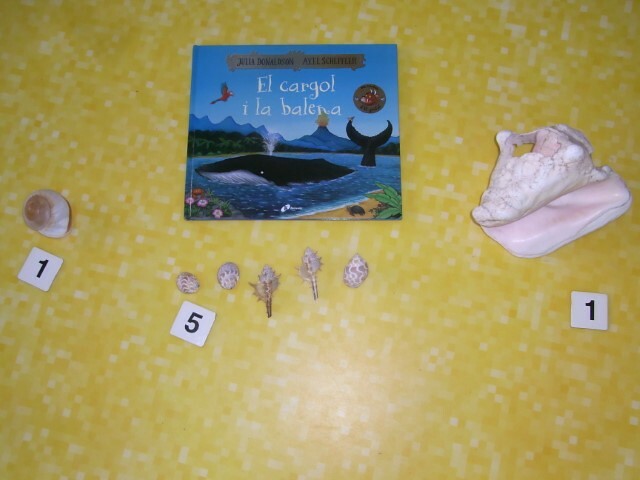This overhead photo captures a meticulously arranged collection of items on a speckled yellow and white tabletop. At the top center of the image, there's a rectangular children's book titled "El Cargo y la Ballena." The book cover features a colorful design with a flying parrot to the left and a blurry badge to the right of the title. The central illustration depicts a baleen whale with water spouting from its blowhole, swimming close to a beach that hosts a crab and some flowers. Below the book, towards the left-center side, lies a roundish shell accompanied by a placard marked with the number 1. To the right of this shell is a series of five smaller shells neatly lined up, with a placard labeled number 5 beneath them. Further to the right-center, there is a larger conch shell, also marked with a placard numbered 1. The entire arrangement rests on a shiny, yellow tabletop that features a grid-like pattern speckled with white, possibly indicative of a kitchen floor or a patterned table surface. The shells vary in color from tan to brown, enhancing the overall aesthetic of the composition.